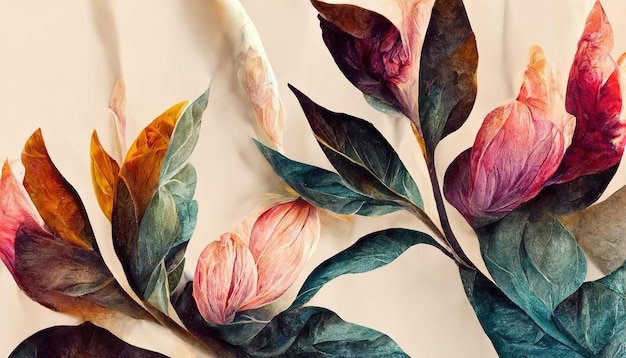The image appears to be an intricate and realistic artwork of several flowers, rendered in a style that is hard to distinguish between a highly detailed painting or a colored pencil drawing. The background is a creamy beige tone that enhances the vividness of the foliage. The flowers, rising up from the bottom, showcase an array of vibrant colors including light pink, dark fuchsia, orange, red, and a subtle purple, with some looking slightly wilted. The accompanying leaves exhibit a spectrum of colors as well, from soft greens and browns to deep blue hues. The composition is rich with varied flora, creating a textured and somewhat three-dimensional effect, particularly noticeable in the distribution of vines and leaves throughout the image. The right side notably features deep fuchsia, green, and brown hues, while the left side contrasts with lighter pinks, oranges, and more greens, giving the piece a balanced yet dynamic visual appeal.